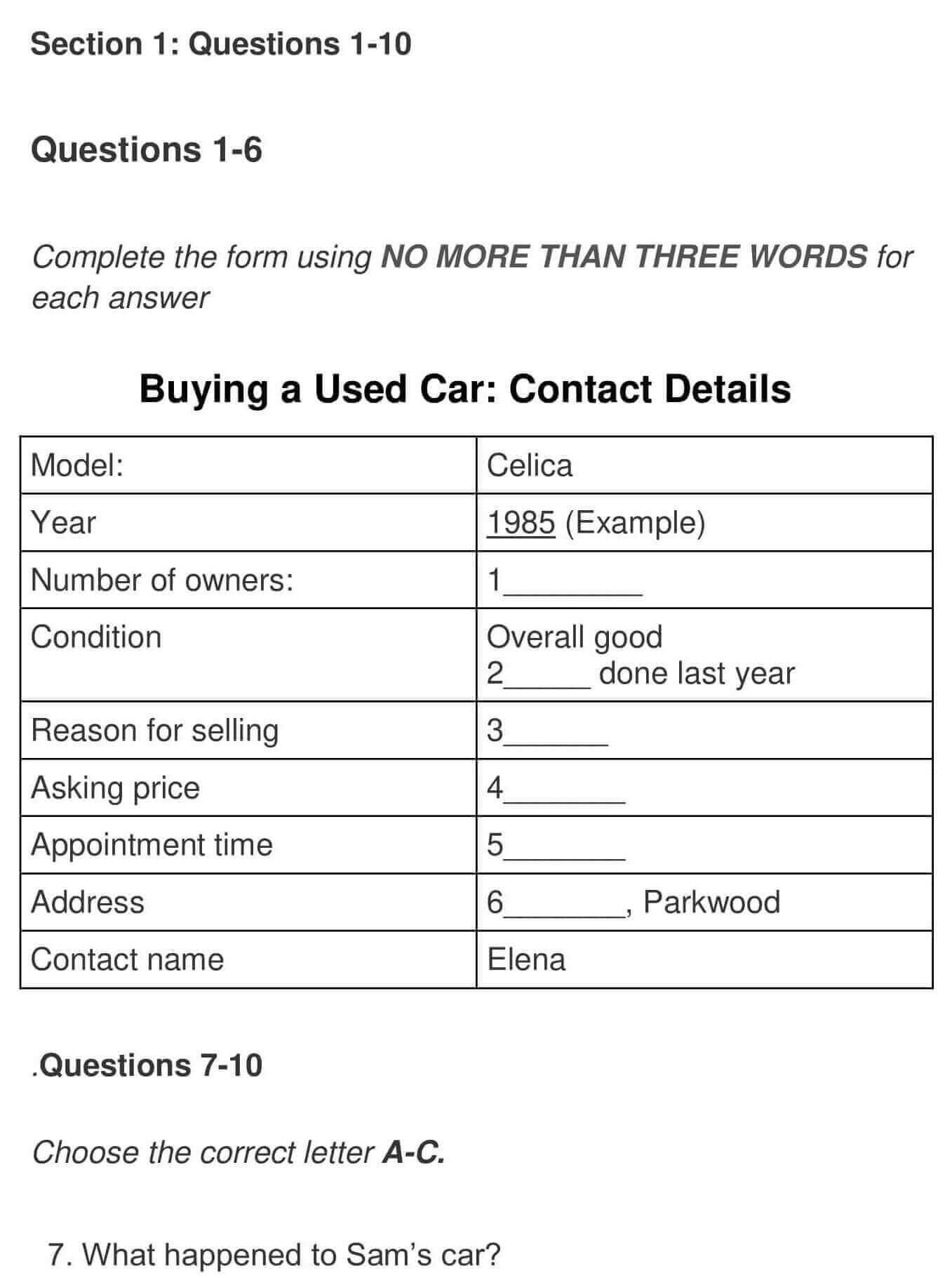The image showcases a detailed black-and-white fill-in document form, likely used for purchasing a used car. The form is neatly aligned with black text on a white background, making it easy to read. At the top, it reads "Section 1: Questions 1-10," with a sub-heading instructing to "Complete the form using NO MORE THAN THREE WORDS for each answer," emphasized in all caps. This is followed by the heading "Buying a used car: Contact Details."

The table beneath has two columns, listing categories on the left and corresponding fields on the right. Some fields are prefilled, while others are blank. The prefilled details include:

- Model: Celica
- Year: 1985
- Number of Owners: One
- Condition: Overall good
- Contact Name: Elena

The remaining fields such as Reason for Selling, Asking Price, Appointment Time, and Address are left blank for the user to fill in. Below the table, sections for questions 7-10 instruct the respondent to "Choose the correct letter A to C." One visible question reads, "What happened to Sam's car?"

Overall, the image displays a well-organized, structured questionnaire meant for facilitating the purchase of a used car, with emphasis on brevity and clarity in the answers.